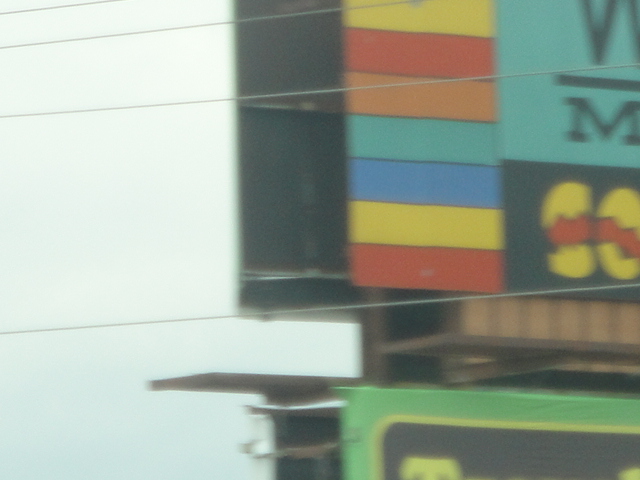The image depicts a large, colorful billboard, likely situated alongside a busy road or highway, evidenced by the visible power lines and the overcast sky overhead. The billboard features a series of uniformly sized vertical stripes in a descending order of yellow, red, orange, aqua, blue, yellow, and red. Adjacent to this striped section, the main part of the billboard is blue with some black lettering which is partially obscured. Below this, a second billboard with a green outline and a black center can be seen, adorned with yellow letters and red accents. A small platform, presumably for maintenance personnel, slightly protrudes from the billboards. The combined elements and the power lines suggest the scene is set along a frequently traveled road.